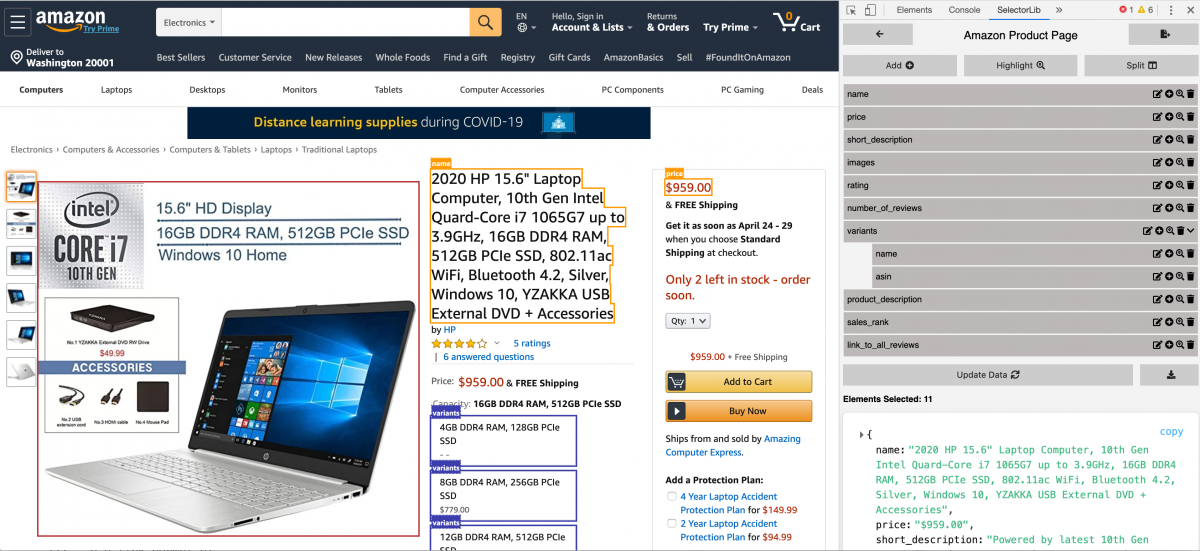This screenshot displays a detailed view of an Amazon webpage. In the upper left-hand corner, the iconic Amazon logo is prominently featured, showcasing the characteristic orange arrow that swoops from left to right. Directly adjacent is a search bar prefilled with the term "electronics," accompanied by a drop-down menu.

To the right of the search bar, users can access their account options through links labeled "Account & Lists," "Returns & Orders," and the option to "Try Prime." The cart, currently empty, is denoted by a large zero in orange.

Spanning the top of the webpage is a black banner alerting users to "Distance Learning Supplies During COVID-19." This banner features a blue box along its length. Below, various categories are listed, including "Computers," "Laptops," "Desktops," "Monitors," "Tablets," "Computer Accessories," "PC Components," and a partially obscured category likely related to events.

Centered on the page is a featured product: an Intel Core i7 10th generation laptop. Detailed specifications are provided: a 15.6-inch display, 16GB of RAM, and Windows 10 Home. The price, prominently displayed in red, is complemented by a vertical lineup of images showcasing the laptop from different angles.

To the right of this first product is another featured listing, possibly for the same laptop, outlined in gold with the price again highlighted in red, and it offers free shipping. Additional purchasing options are indicated with purple boxes. A notification shows there are only "two left in stock," urging shoppers to "order soon." Options to add the item to the cart or to buy immediately are also displayed.

Further to the right is an additional Amazon product section, listing different, likely older products against a gray background.